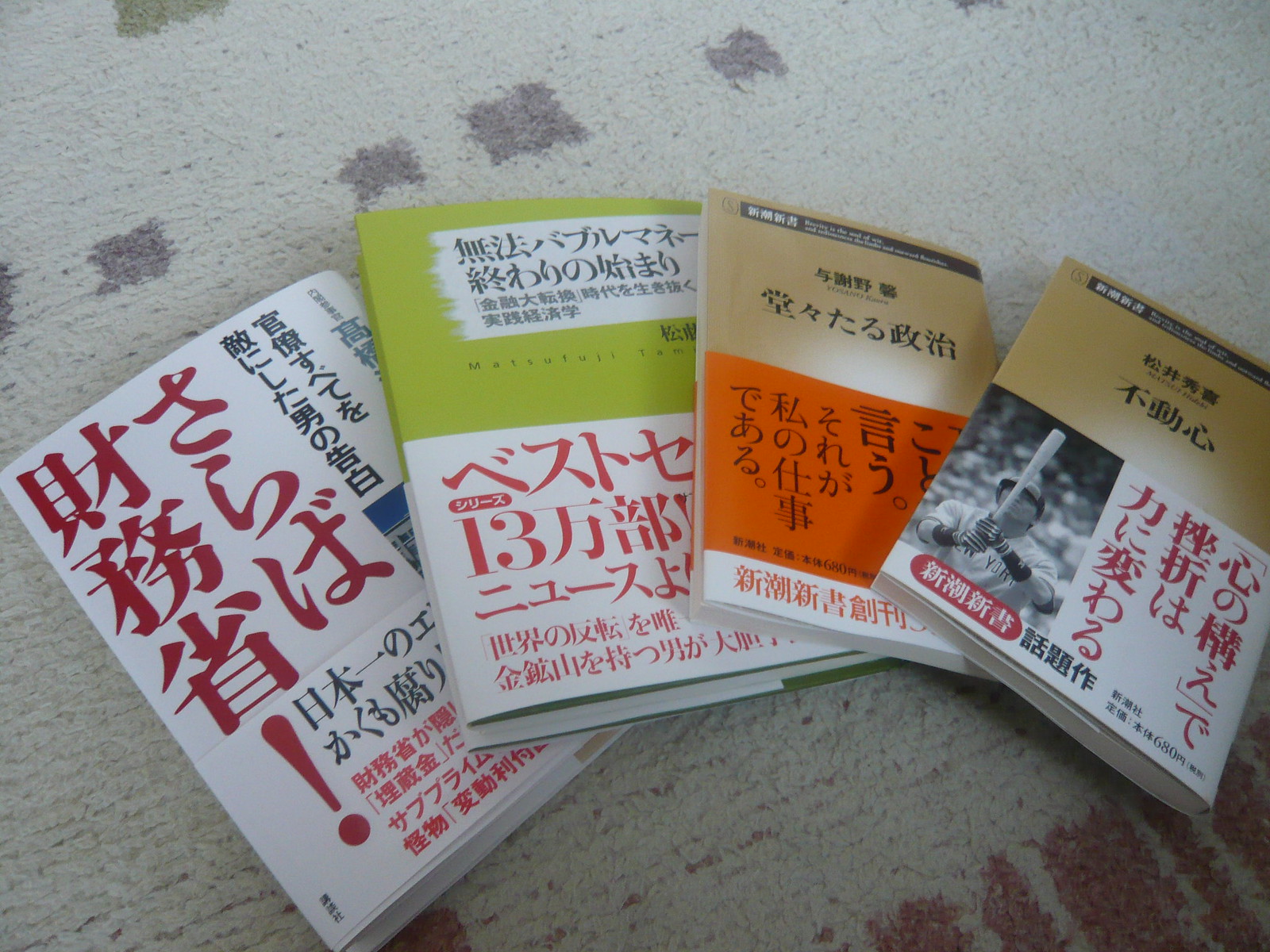This is a detailed color photograph featuring four Asian paperback books, specifically with text in Japanese and/or Chinese, arranged in a fanned-out manner on a textile surface. The surface appears to be a whitish or off-white hand-knit blanket, featuring distinct red threads and purple boxes. The covers of the books predominantly use white as a background, adorned with a mix of black and red text. Notably, the top section of one book is light green, while the bottom section of another is orange. One of the books displays a black-and-white photograph of a professional New York baseball player. The books overlap slightly but are clearly distinguishable, positioned neatly on the textured blanket.